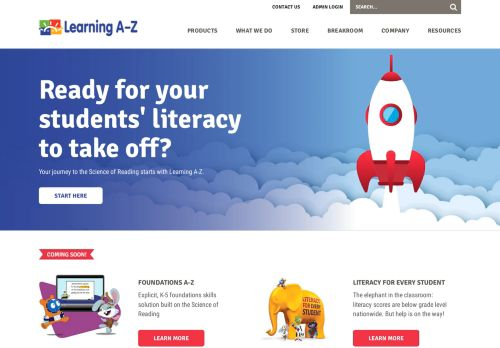The image depicts an educational website called Learning A to Z. The logo, reminiscent of the classic Windows logo with its four colorful panes—green, red, blue, and yellow—is creatively reimagined with a half-sun illustration in white, giving it a unique, tilted appearance. The page shown appears to be a launch page featuring a graphic of a rocket ship soaring above the clouds, accompanied by the text: "Ready for your students' literacy to take off. Your journey to the source of learning starts with Learning A through Z. Start here." The text is small and somewhat illegible due to noticeable JPEG compression artifacts. 

At the top of the page, the navigation menu includes options such as Products, What We Do, Store, Break Room, Company, and Resources, along with a search bar. Toward the bottom of the page, two sections are highlighted: "Foundations A through Z," featuring an image of a laptop and two cartoon characters, and "Literacy for Every Student," illustrated with a golden elephant. The detailed descriptions within these sections are difficult to read. The website's design evokes a mid-2000s aesthetic, lacking modern elements like a hamburger menu, suggesting it may be slightly outdated despite possibly recent origins.